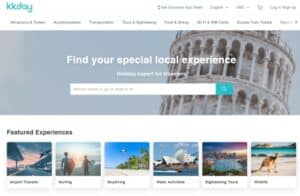The image appears to be a low-resolution screenshot or mock-up of a travel website on a white background. The top left corner features a blue, illegible logo. Below the logo, there is text composed of a combination of longer words and shorter phrases. The navigational menu consists of eight options in either white or black text on a white background, with the rightmost menu item potentially offering a dropdown functionality.

Below the menu, there's a photograph capturing a close-up view of the Leaning Tower of Pisa during daylight, positioned to the right. Overlaying the image is white text that reads, "Find your special local experience," adjacent to a text input box and a blue search button.

Under this section, the phrase "Featured Experiences" introduces a gallery of six images, each accompanied by brief, single-line captions. Despite the low resolution, the images depict various vacation destinations, including urban landscapes, beach scenes (morning and afternoon), mountainous regions, an aerial view of a resort, and a child playing with a sandcastle on a beach.

Overall, this caption provides a thorough description of the elements and layout of what seems to be a travel-themed website, despite the clarity limitations of the original image.